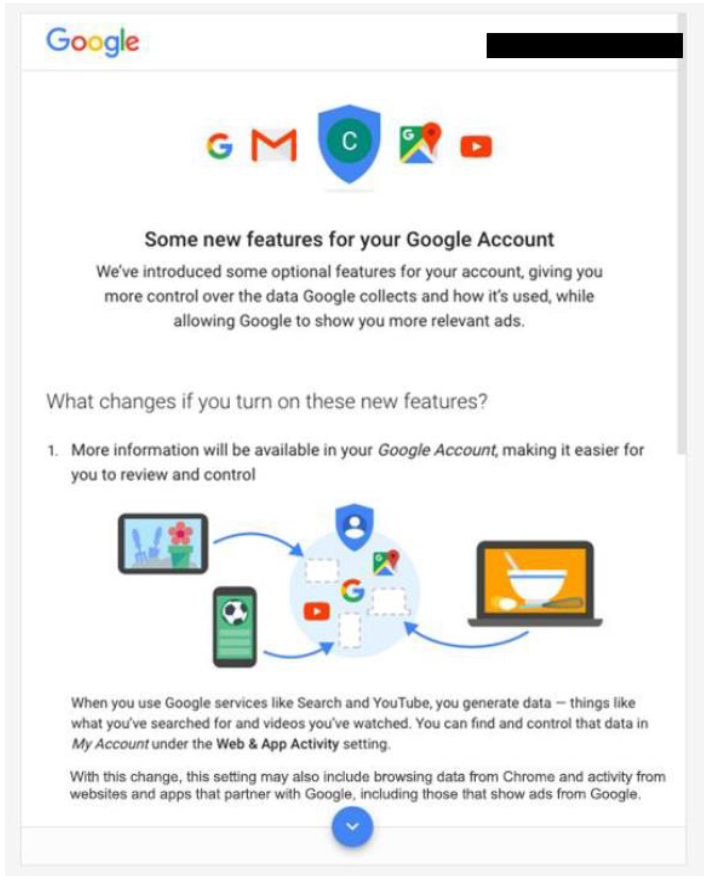Sure, here’s a detailed and cleaned-up descriptive caption for the image:

---

The image is a screenshot demonstrating several features available within Google Apps. At the top, it displays a row of recognizable Google icons: the Google G logo, an email envelope, a shield with the letter 'C', the Google Maps pin, and the YouTube red play button.

Below the icons, a prominent black text reads, "Some new features for your Google account." This introduction mentions that Google has introduced optional features aimed at giving users more control over the data collected and delivering more relevant ads.

Further down, there’s a section titled, "What changes if you turn on these new features?" followed by an explanatory note that turning on these features will provide more accessible and manageable information within one's Google account.

A graphic near this text illustrates various devices pointing towards a central circle containing a shield icon with a human silhouette, symbolizing data security and user control.

Lastly, additional informative text explains how using Google services like Search and YouTube generates data that can be reviewed and controlled in "My Account" under the "Web and App Activity" setting. This setting could also include browsing data from Chrome and activities from partner websites and apps that show Google ads. At the bottom, there's a small blue circle with a downward-pointing white arrow, indicating further options or information.

---